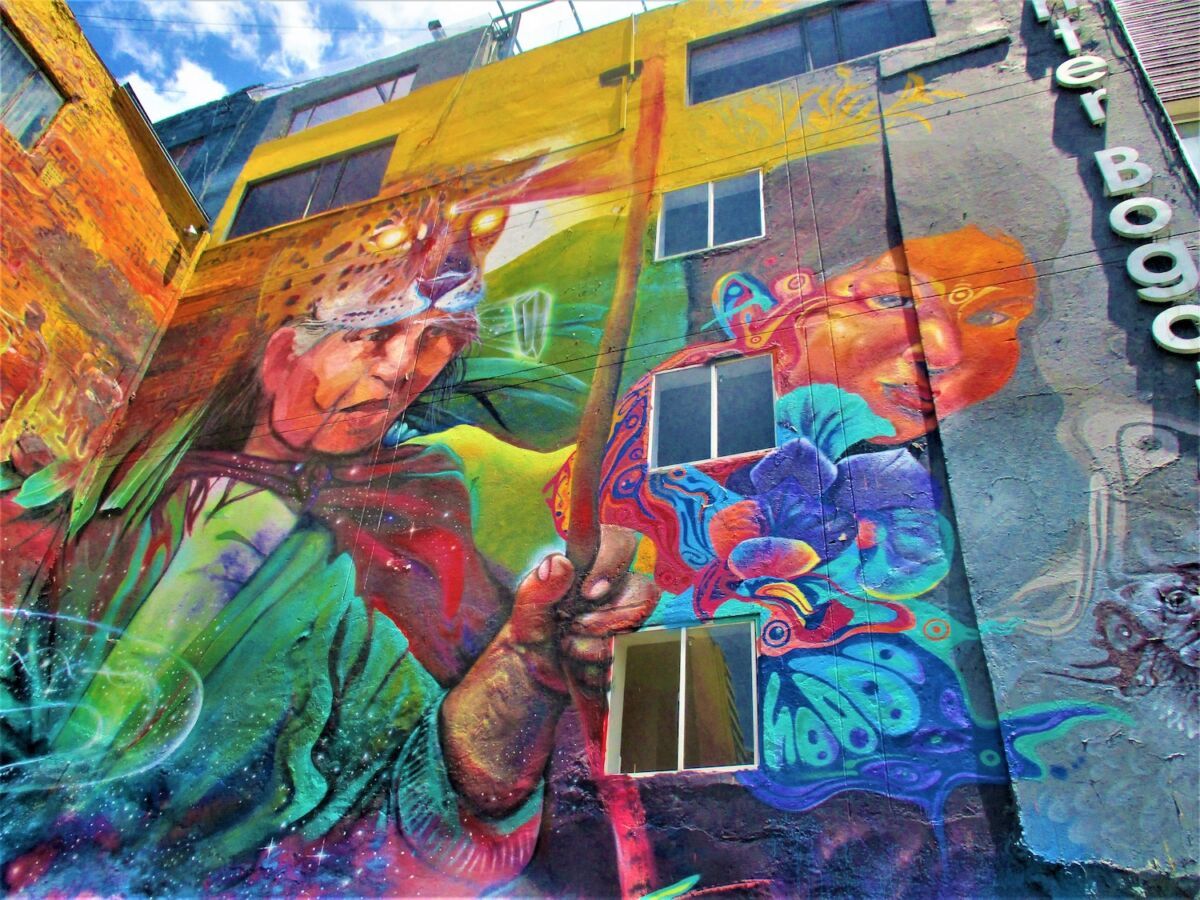The photograph captures an expansive, multi-story building set in an urban environment, possibly within a large town or city, on a somewhat cloudy day. The image is square, vividly colorful, and brimming with details. At ground level, an intriguing and imaginative mural sprawls across the building's exterior. The mural features two primary figures: on the left, a male warrior donning a green cloak, a red and burgundy shirt, and a striking leopard skull helmet with glowing yellow eyes. He is wielding a wooden spear or staff. On the right, a woman adorned in a vibrant ensemble of blue, purple, and orange, with blue feathers in her thick brown hair and a golden circle on her forehead. Her face is a warm, orangish-brown hue. The mural's background is a lively mix of bright yellows and greens, punctuated by an incomplete text reading "T-E-R B-O-G-O" in the upper right corner. Decorated with a large blue, purple, and red flower, the mural adds a burst of creativity and color against the building's gray facade, capturing the essence of urban street art and indigenous imagery.